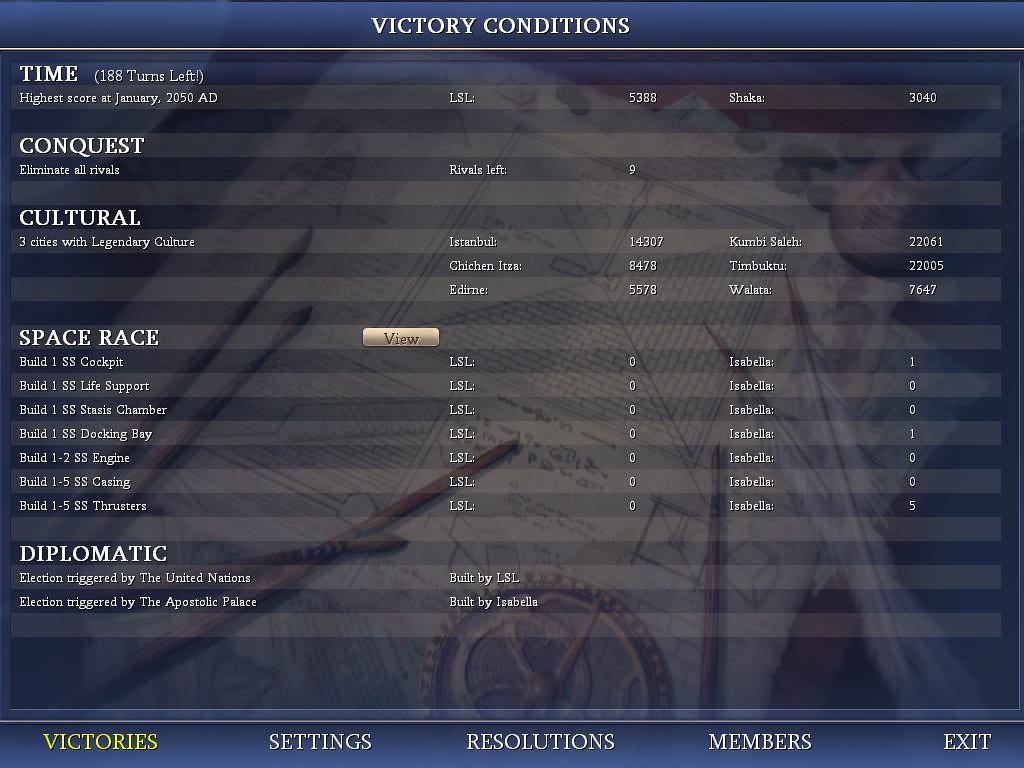The rectangular image appears to be a screenshot from a video game, featuring an old-school, artistic background with drawings, a compass, paintbrushes, and feather quills reminiscent of historical writing tools. Overlaying this intricate backdrop is a predominantly blue chart titled "Victory Conditions." The chart lists categories such as Time (with details like "188 turns left" and the "Highest score at January 2050 AD"), Conquest ("eliminate all rivals" with "9 rivals left"), Cultural ("3 cities with legendary culture"), Space Race (with various builds), and Diplomatic specifications. The left-hand side of the chart lists these headings, while detailed information is charted to the right. At the bottom of the screen, there are several tabs labeled Victory, Settings, Resolution, Members, and Exit, with the "Victory" tab highlighted in yellow. The overall impression is a user interface from a video game, likely viewed on a computer or console, combining both strategy and detailed progress tracking.